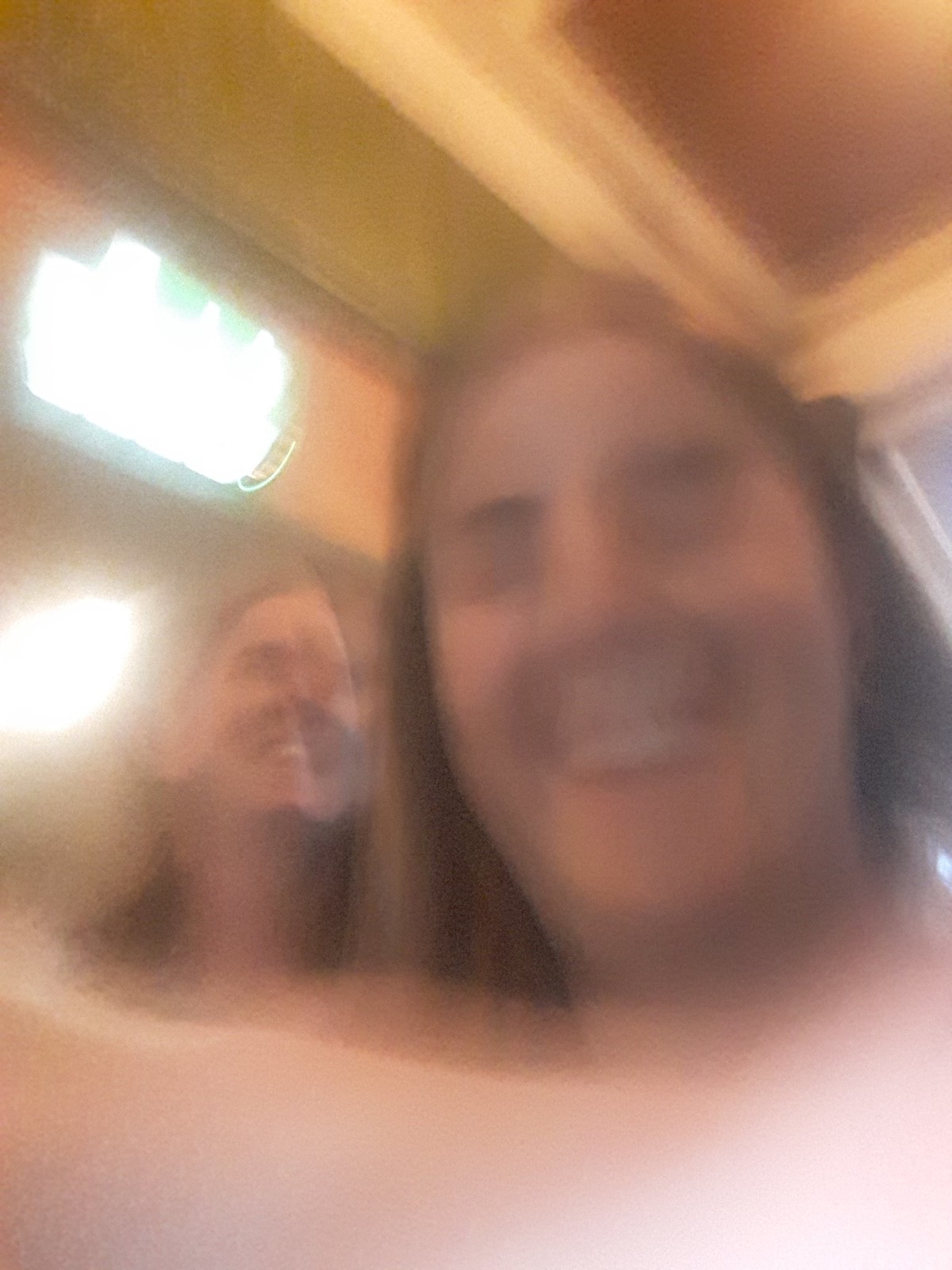The image captures a close-up of a girl with long brown hair, joyfully laughing with her eyes closed. Her face dominates the frame, and her teeth are visible in her broad smile. The setting is somewhat ambiguous, suggesting she might be inside a vehicle or a structure with a wooden trapdoor-like feature above her head. To her left, another girl is also laughing, her eyes directed upwards, exposing her teeth as well. The second girl is positioned in front of a cutout in the wall, through which a bright sky and two hanging leaves are visible. Further behind, there's another window allowing additional light into the scene. The wooden elements around them hint at a crawl space above, although the setting remains difficult to definitively identify due to the image's blurriness.